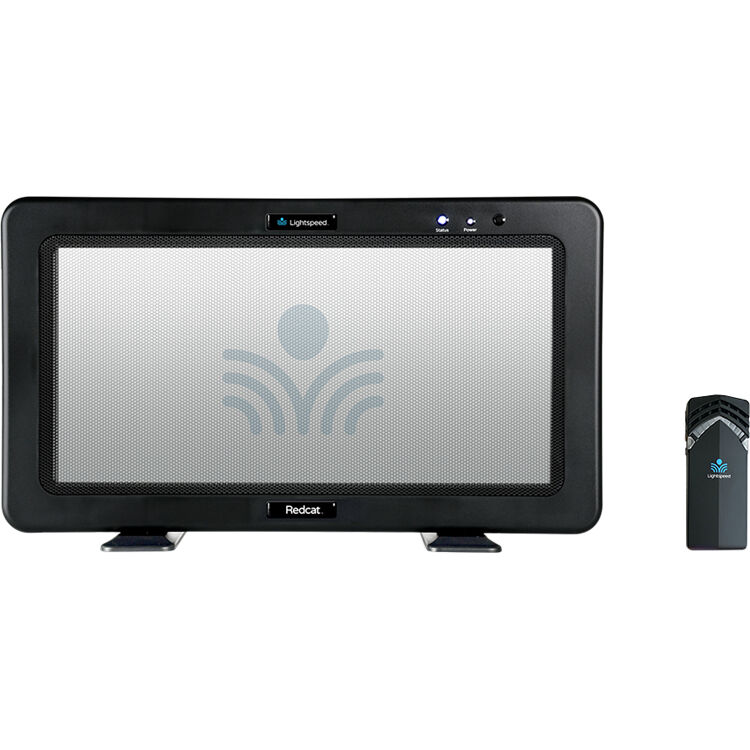The image features a rectangular video screen with a black plastic border and short legs, resembling that of a TV set. The screen, which has a white background, prominently displays a simple pale gray logo consisting of a circle, a V-shape beneath it, and two curvy lines on each side. At the top of the border, there's a black placard with the word "Lightspeed" written on it accompanied by a blue icon. Below the screen, another placard bears the name "Red Cat" in white text on a red background. The screen's black edge houses three buttons, one of which is clearly labeled "Power." To the right of the screen, there is an image of a black remote control device, devoid of numerical labels.